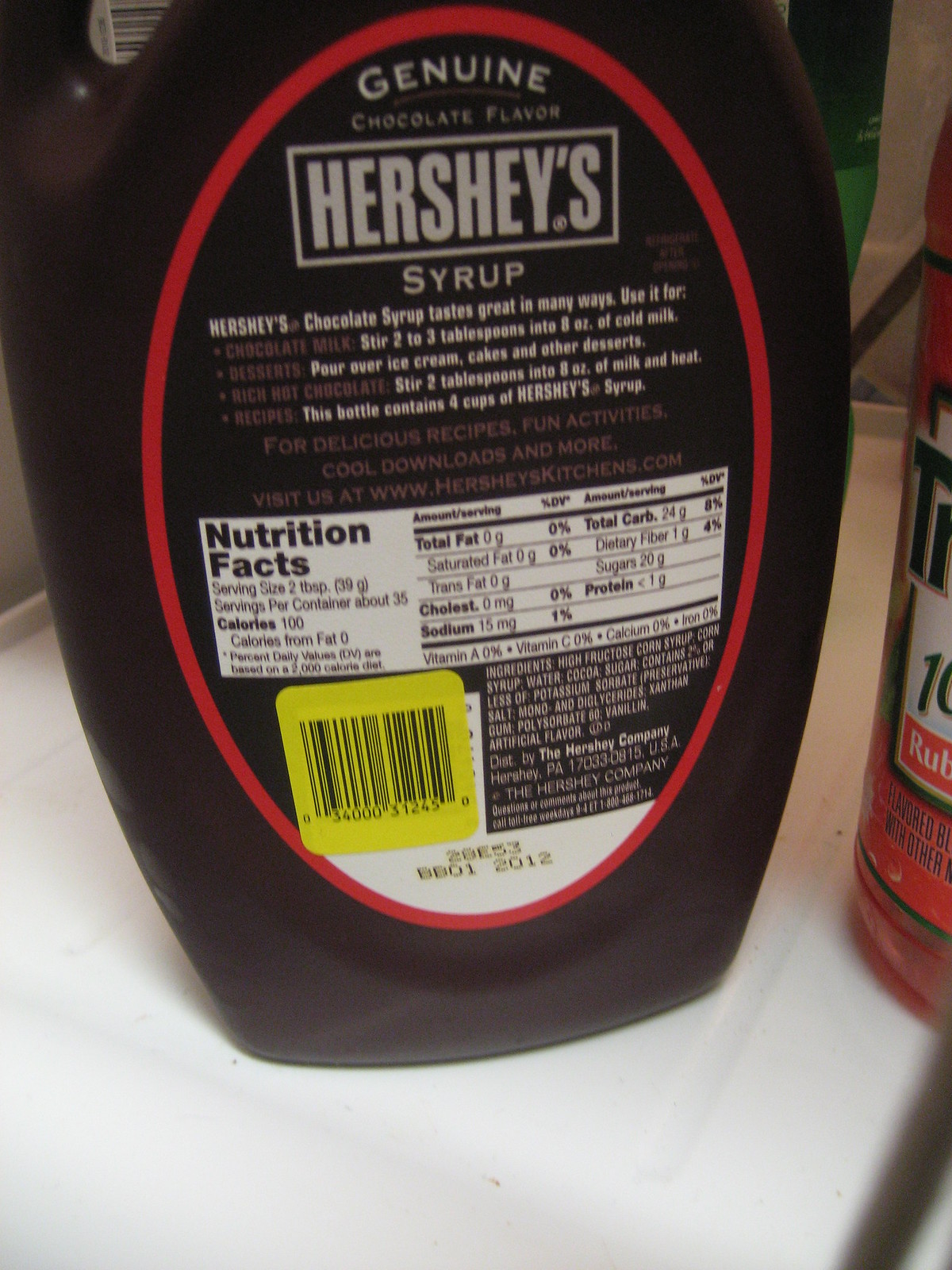This rectangular image captures a close-up photograph of a large Hershey’s syrup container placed on a white counter or table. The container fills approximately three-fourths of the frame, prominently showcasing the back label from nearly the bottom to close to the top, though the spout is not visible. The label, bordered in red, prominently reads "Genuine Hershey's Syrup." It elaborates that Hershey's chocolate syrup is versatile and delicious, ideal for chocolate milk, desserts, rich hot chocolate, and various recipes. Additionally, the nutritional facts are listed: the container holds about 35 servings, with each serving size being two tablespoons and containing 100 calories, 0 grams of total fat, 24 grams of total carbohydrates, and 15 milligrams of sodium. At the bottom of the label, the best-before date is noted as "01-2012," and the lower-right corner indicates that the product is distributed by The Hershey Company, based in Hershey, Pennsylvania, USA.